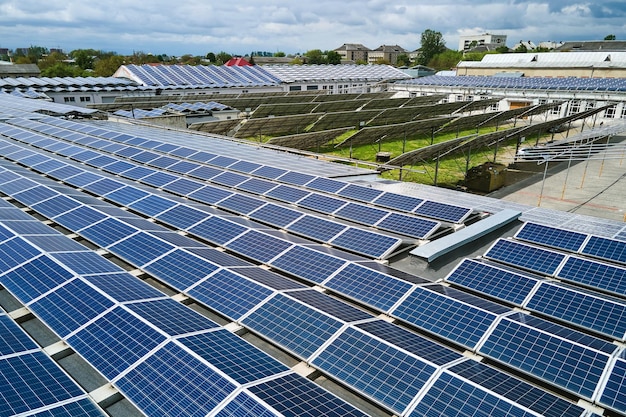The image is a color photograph taken outdoors on a sunny day, featuring a vast array of solar panels. The entire scene is filled with solar panels of various sizes, positioned at different angles and covering a roof or platform. The panels, framed in white and dark blue in color, form a distinct V shape at the bottom of the image, converging at a point. In the center area, some panels are turned away, making their fronts less visible. Additionally, there is a green grassy area amidst the solar panels, visible further up in the image. The top section reveals more solar panels, along with several tall buildings, greenery, and trees. Blue sky and large, billowy clouds dominate the background, highlighting the sunny environment. The entire scene captures the expansive setup of solar panels bathed in sunlight with no people present.